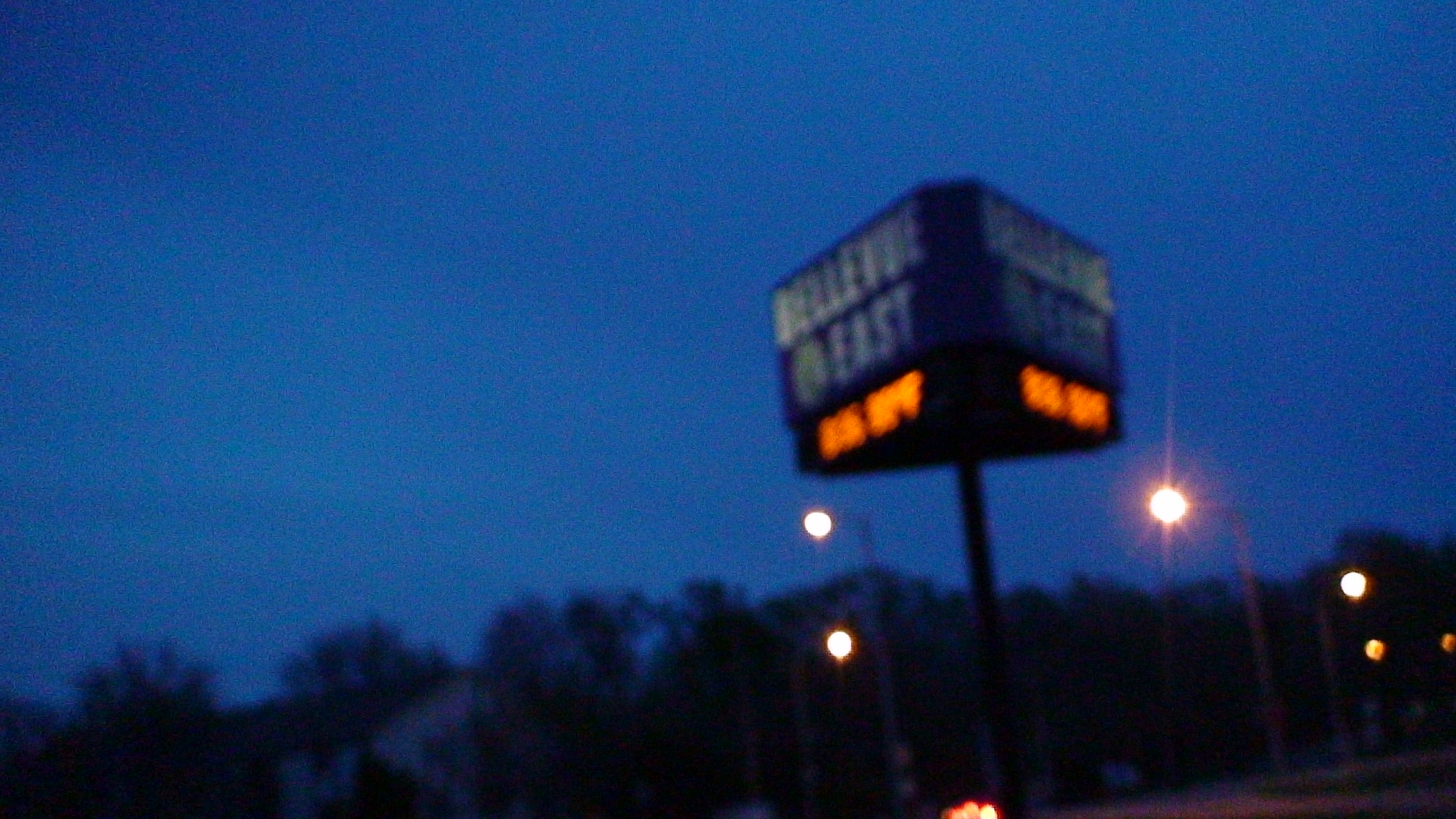In this image, we observe a large, rotating sign with a triangular cube shape, featuring multiple sides that display the same text. Captured late at night, the image suffers from significant blurriness, making it difficult to discern the exact wording on the sign. The sky in the background is nearly black, adding to the dim ambiance. The sign has a dark blue background with an all-white logo prominently displayed. Below the blue section, there is a black area adorned with neon orange text, though the blur obscures the specifics. Additionally, some streetlights are visible in the background, providing limited illumination against the dark night.